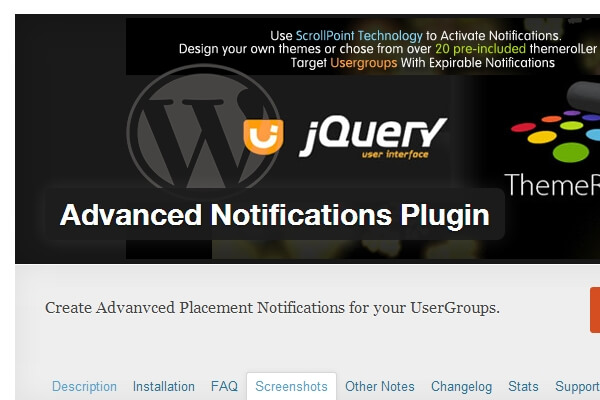### Descriptive Caption:

The image appears to be a sophisticated webpage design or a UI mockup encompassing various elements related to notification technology and customization. 

Central to the design is a dark gray rectangle featuring text that explains key functionalities. It reads: "Use Scroll Point Technology to activate notifications. Design your own themes or choose from over 20 pre-included thermo lit target user groups with expirable notifications." The majority of this text is in a clean white font. Notably, "scroll point technology" is highlighted in blue, "20 pre-included" in green, and "user groups" in orange.

Above this informative block, there is a distinct logo: a stylized 'W' in a serif-like font, black in color, but crafted as a knockout, revealing a gray circle cutout within it. 

Further down, there is another striking visual—depiction involving a smiley face-like design element resembling a 'U' with a cut in it, displayed in white over a black and orange shield. Below this, the term "JQuery" is prominently displayed, followed by the description "User Interface," suggesting a focus on advanced web technologies.

Decorating the design are several multicolored circles—purples, oranges, blues, greens, yellows, and reds—adding vibrant accents across the layout.

In another section, the phrase "Advanced Notification Plug-in" stands out, followed by a message encouraging users to "create advanced placement notifications in your user groups."

A navigational menu is visible, featuring various tabs: "Description," "Installation," "FAQ," "Screenshot," (highlighted), "Other Notes," "Channel," "Change Log," "Stats," and "Support," indicating a comprehensive set of resources and support options for users.

Overall, the design conveys a high level of detail and functionality, geared towards providing customizable and advanced notification solutions.